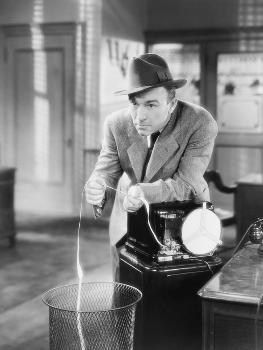In this black-and-white photograph set in the 1930s or 1940s, a man donning a detective-style hat and a suit stands prominently. He gazes intently at something off-screen while holding a long string that appears to lead into a woven wastebasket in front of him. His arm rests on a black post, and the background is detailed with a door, several windows adorned with silhouettes of blinds, and partial reflections of light. Beside him, a granite-topped table holds part of a telephone, and a glimpse of an office chair is visible. The setting evokes an old-time office environment, with the man seemingly engaged in a focused task involving the string, potentially related to a period-specific device or machinery.